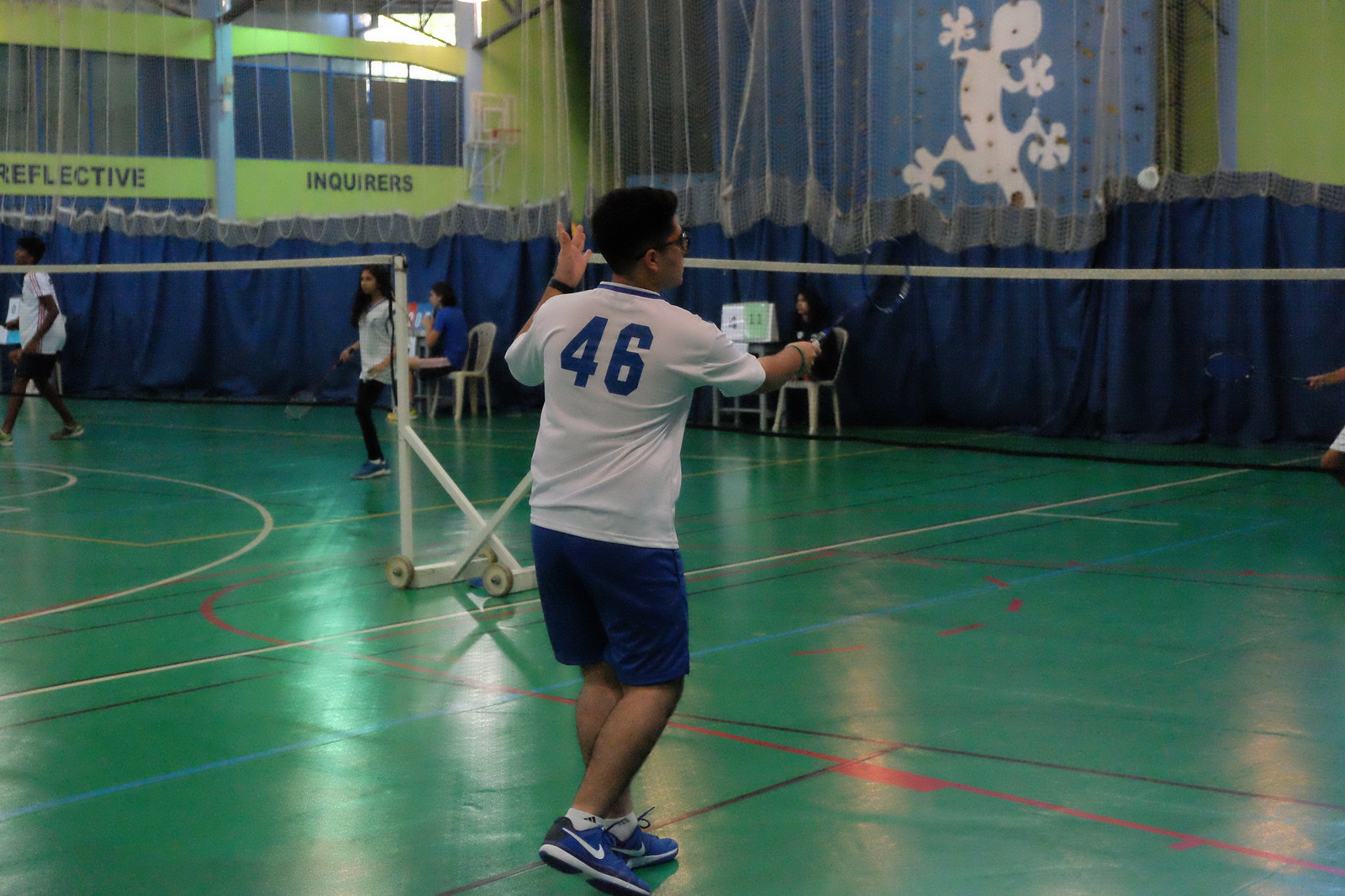The photograph captures the interior of a gym featuring two adjacent green badminton courts marked with red, yellow, blue, and white lines. A curtain with a blue bottom and clear top hangs about 25 to 30 feet high in the background. On the left court, two women are engaged in a badminton game, with two more women seated in plastic chairs behind them. The right court shows a man, seen from behind, playing badminton. He has dark hair, wears glasses, and is dressed in a white jersey with a blue number 46, blue shorts, white ankle socks, and blue Nike shoes with a white stripe. The gym's walls display an inscription reading "Reflective Inquirers," adding to the ambiance of the scene.